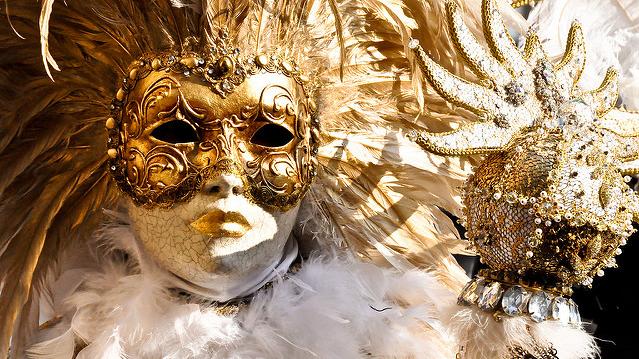The image is a vibrant and detailed color photograph in landscape orientation showcasing a person adorned in an elaborate, festive costume. The focal point is a woman wearing a striking, full-face golden mask, intricately decorated with beads, ornate designs, and sparkling trims, emphasizing her eyes and lips with more gold accents. Surrounding her head is an impressive fan of feathers, primarily gold but complemented with white ones forming a collar beneath her chin. Her eyes appear dark and slightly mystical behind the small cutouts of the mask.

In her right hand, she holds a small, intricately detailed jester-like ornament, which is adorned with white gems and pin-like pearls, further enhancing the festive, Mardi Gras-like ambiance with its splendid embellishments.

On her arm, there is a golden accessory, resembling a jeweled orb with a crest-like, sunburst top, encrusted with beads and pointy details all around it. This opulent costume, laden with various sparkling elements and richly decorated feathers, reflects the celebratory spirit of events like Mardi Gras, captured in a style that blends realism with representational art.